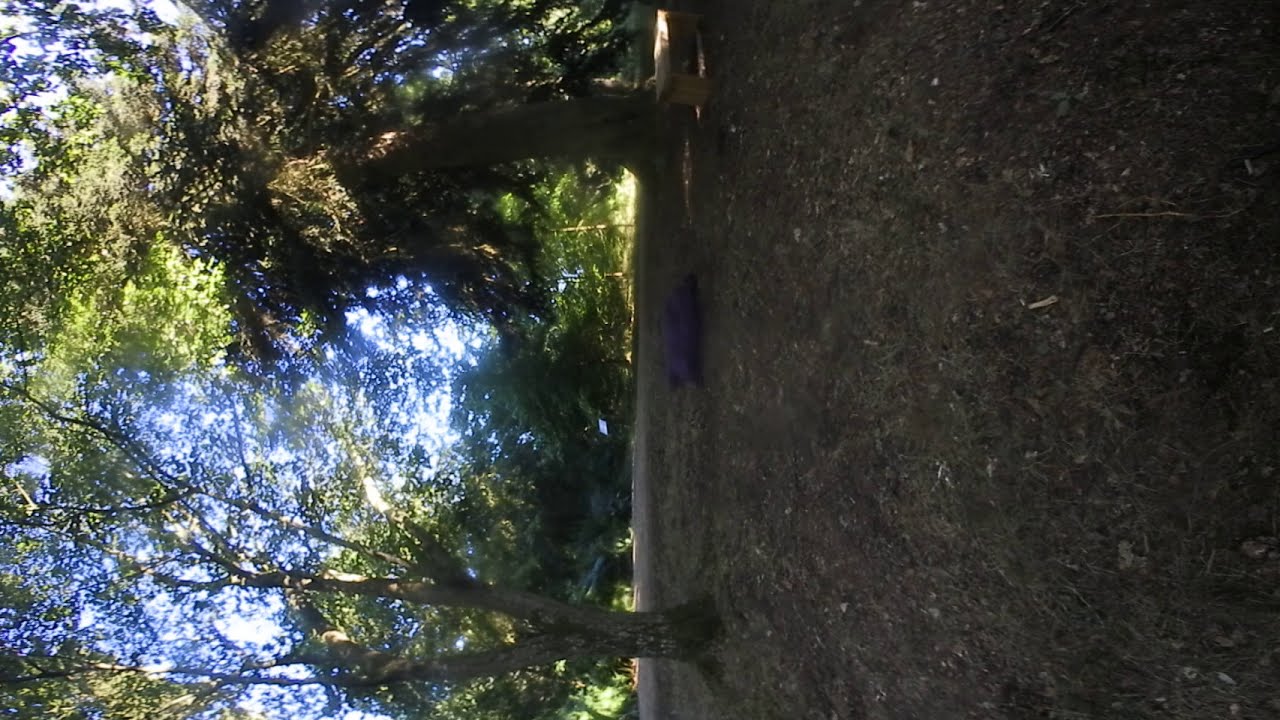This image is a clear, high-definition photograph taken outdoors, showing a serene and vibrant natural setting. The image appears to be sideways, with two prominent trees in the foreground against a barren dirt hillside covered sporadically with grass and sticks. The tree closest to the bottom has a narrow trunk that branches into two larger trunks, adorned with light green leaves concentrated mostly at the top. The adjacent tree features a much thicker single trunk with leaves that are a rich combination of dark green and brown. Between these trees, there's an indistinct object that resembles a rock, log, or perhaps a purple pillow. Beyond the foreground, a grove of trees with various shades of green forms the background, interspersed with glimpses of a light blue, cloud-speckled sky. Shadows cast across the image suggest it's late in the afternoon, around four o'clock, highlighting the contrast between the barren foreground and the lush greenery above, catching the sunlight in a picturesque manner. The vivid colors and crisp detail make this natural scene quite striking.